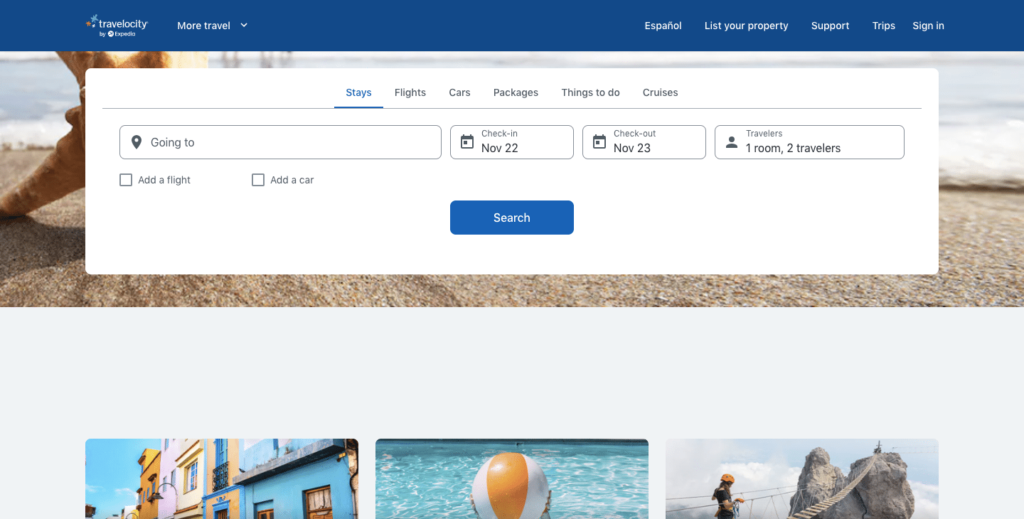The top left corner displays the Travelocity logo, signaling that this is a travel website. Below, there are options for "More Travel" and a blue rectangular button labeled "Español." The navigation menu includes links for "List Your Property," "Support," "Trips," and "Sign In." Below, there are additional tabs for "Stays," "Flights," "Cars," "Packages," "Things to Do," and "Cruises."

A red square prompts users with fields labeled "Going to," "Check-in," "November 22," "Check-out," "November 23," and "Travelers: 1 Room, 2 Travelers." Options to "Add a flight" or "Add a car" are also available. A blue square labeled "Search" serves as the call-to-action button.

In the background, a picturesque beach scene unfolds with clear blue waters and sandy shores. There’s a person visible in the landscape, standing on what appears to be dirt. In the bottom left, vibrant, colorful buildings add a splash of charm. An inflatable ball floats in a nearby pool of water. To the right of the pool, a bridge extends across the scene with rope handrails, appearing somewhat precarious.

The sky is dotted with white clouds, adding to the idyllic setting of this comprehensive travel planning webpage.